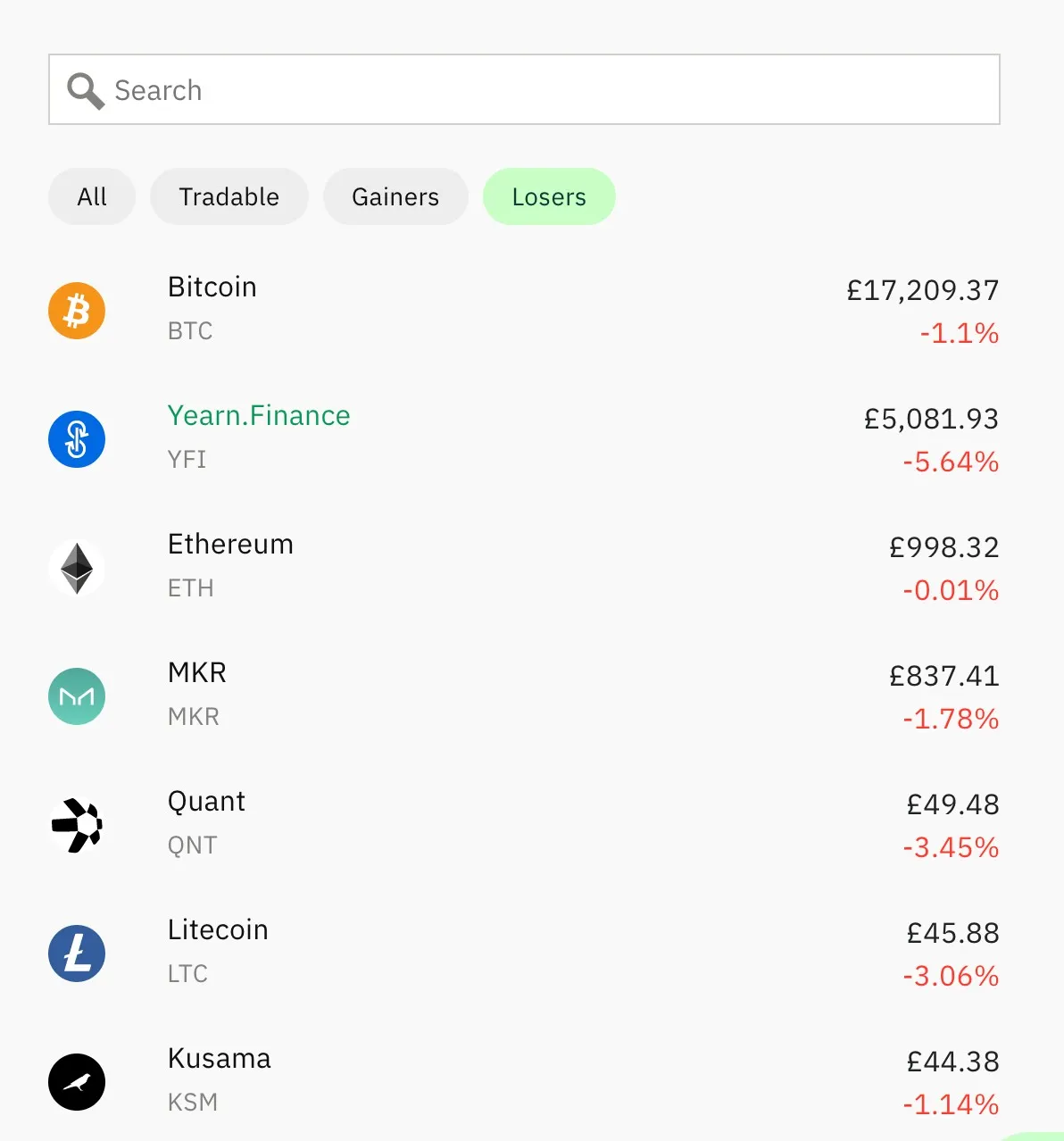This is an image of a cryptocurrency trading website interface. At the top of the page, there is a search bar for users to find specific cryptocurrencies. Just below the search bar, there are several tabs labeled "All," "Tradable," "Gainers," and "Losers." The "Losers" tab is currently selected, evidenced by its green highlight. Displayed prominently under this tab is a list of cryptocurrencies that have decreased in value. Each entry on the list includes an icon representing the cryptocurrency, its abbreviation, and its current price in euros. Additionally, it shows the amount of value each cryptocurrency has lost. Notably, Bitcoin is featured among the losers on this page.